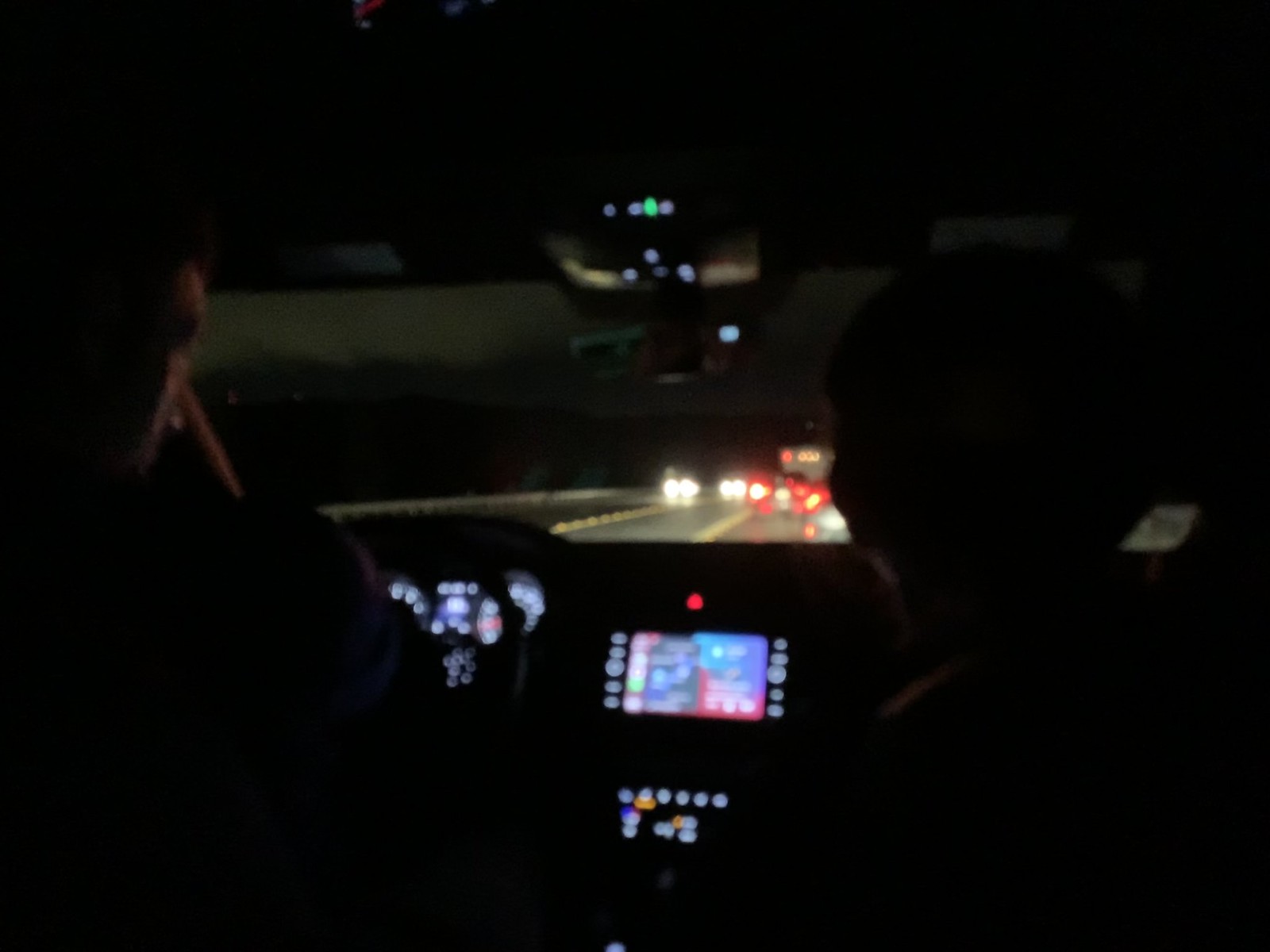The photograph captures a nighttime scene inside a car, viewed from the back seat. Two people are seated in the front; the driver appears to be an adult male, and the passenger is likely a young boy. The vehicle's interior is dimly lit, with the dashboard and center console illuminated by various displays and instruments. The most prominent feature is a large central screen flanked by glowing buttons, topped by a red triangle-shaped indicator. Two analog speedometers, with a digital display between them, are also lit up. Outside the car, the scene depicts a busy freeway with the red brake lights of vehicles ahead and the headlights of oncoming traffic visible in the distance. The dark, possibly cloudy sky adds to the overall somber ambiance of the setting.